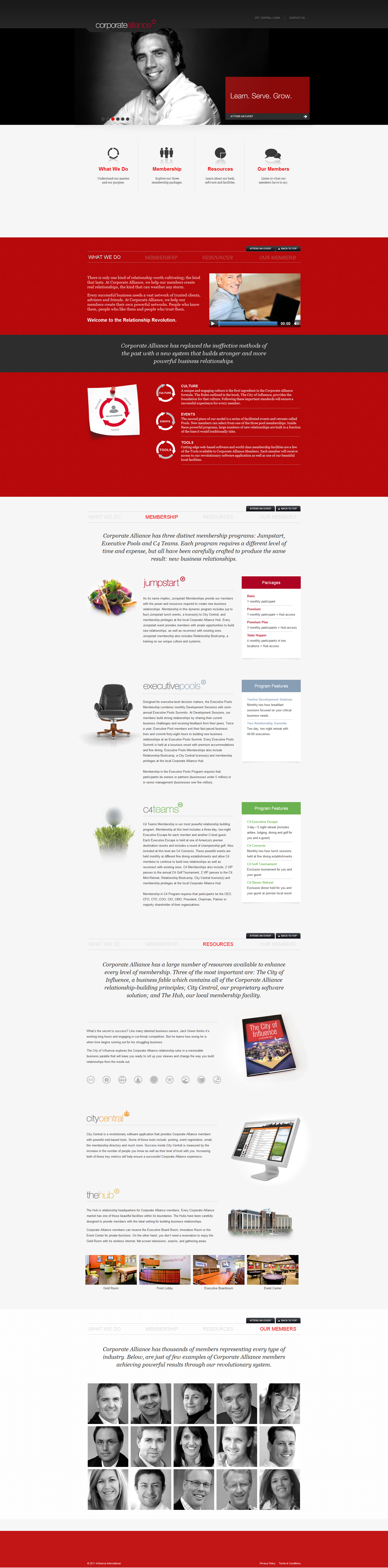This screenshot, originating from an unknown source, bears a dynamic mix of text and imagery aimed at introducing and promoting Corporate Alliance. 

At the top, a striking black-and-white photograph captures a man smiling directly at the camera. He is dressed in a light-colored, collared button-down shirt, exuding a friendly and approachable demeanor. Adjacent to this photograph, the words "learn, serve, grow, attend an event" are prominently displayed.

In the upper left corner above the man's head, "Corporate" is inscribed in white letters, followed by "Alliance" in bold red. 

Beneath the photograph, several sections unfold what Corporate Alliance offers:
- **What We Do**: "Understand our passion and our purpose."
- **Membership**: "Explore our three membership packages."
- **Resources**: "Learn about our book, software, and facilities."
- **Our Members**: "Listen to what our members have to say."

Directly beneath this information is a vivid red banner proclaiming, "What We Do," alongside a powerful quote: "There's only one kind of relationship worth cultivating, the kind that lasts." The banner elaborates on Corporate Alliance's mission to foster enduring, trustworthy business relationships, underscoring the necessity of a robust network for sustained business success.

To the right, a screenshot from a video features an older white man smiling at the camera, an open laptop beside him. Centered below this image is a black banner with white text that delivers a compelling message on Corporate Alliance's evolved approach to building business relationships.

Highlighted next are three core elements of Corporate Alliance's model:
- **Culture**: "A unique and engaging culture based on the rules outlined in 'The City of Influence.'"
- **Events**: Facilitated events and retreats called "pools," where new members can rapidly develop numerous new relationships.
- **Tools**: Advanced web-based software and world-class membership facilities, offering members access to innovative tools and beautiful local facilities.

The final section describes the three distinct membership programs offered by Corporate Alliance:
- **Jumpstart**
- **Executive Pools**
- **C4 Teams**

Each program varies in terms of time and financial commitment but is meticulously designed to cultivate new business relationships. 

This comprehensive layout illustrates Corporate Alliance’s dedication to nurturing and enhancing business networks through culture, events, tools, and tailored membership programs.